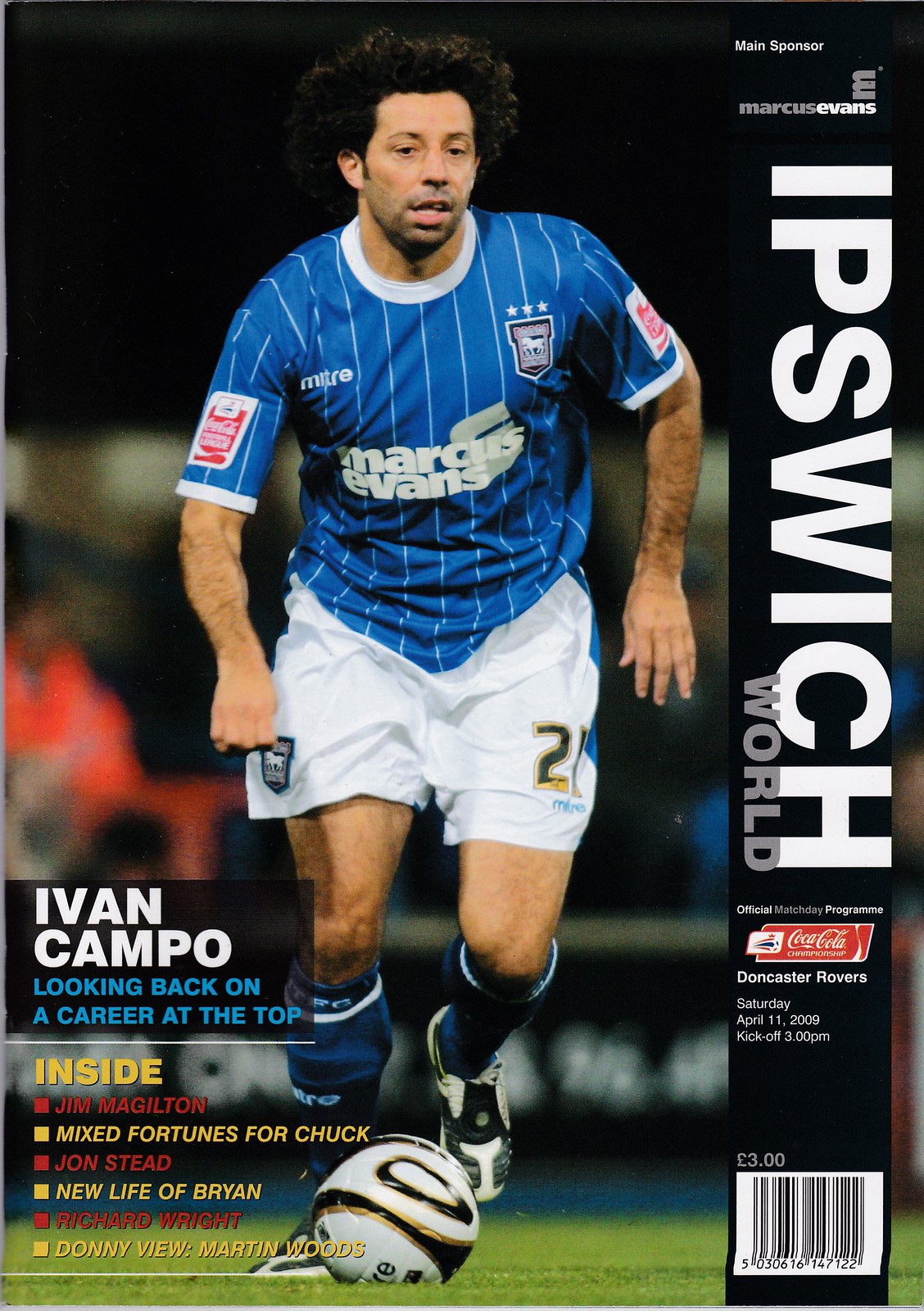The image is a magazine cover featuring a soccer player who takes up nearly the whole image, from top to bottom. The soccer player is mid-run, about to kick a white and black soccer ball with gold accents. He has dark curly hair and light brown skin, and he is dressed in a blue jersey with a white logo in the center, thin white stripes running vertically, white shorts marked with the number 21, blue socks, and white and black cleats. The Coca-Cola logo can be seen on each arm of his jersey. He stands on a bright green soccer field.

In the background, which is blurred with black, white, and orange patches, a prominent black bar runs vertically from the top to the bottom of the image near the right side. On this bar, "Ipswich World" is written in large white capital letters, with "world" in gray letters underneath. Additional details on the black bar include: "Main Sponsor Marcus Evans," "Official Match Day Programs," "Doncaster Rovers, Saturday, April 11th, 2009, kickoff, 3 p.m.," and a barcode in the bottom right corner with "£3" above it.

Inscribed over the image in a semi-transparent black box near the bottom left corner, it reads "IVAN CAMPO" in bright white capital letters, followed by "looking back on a career" in smaller blue letters. Below this and outside the black box, other text descriptions appear: "INSIDE" in yellow letters, followed by a series of names and captions: "Jim Magleton" in red, "mixed fortunes for Chuck" in yellow, "John Stead" in red, "new life of Brian" in yellow, "Richard Wright" in red, and "Donnyview Martin Woods" in red.